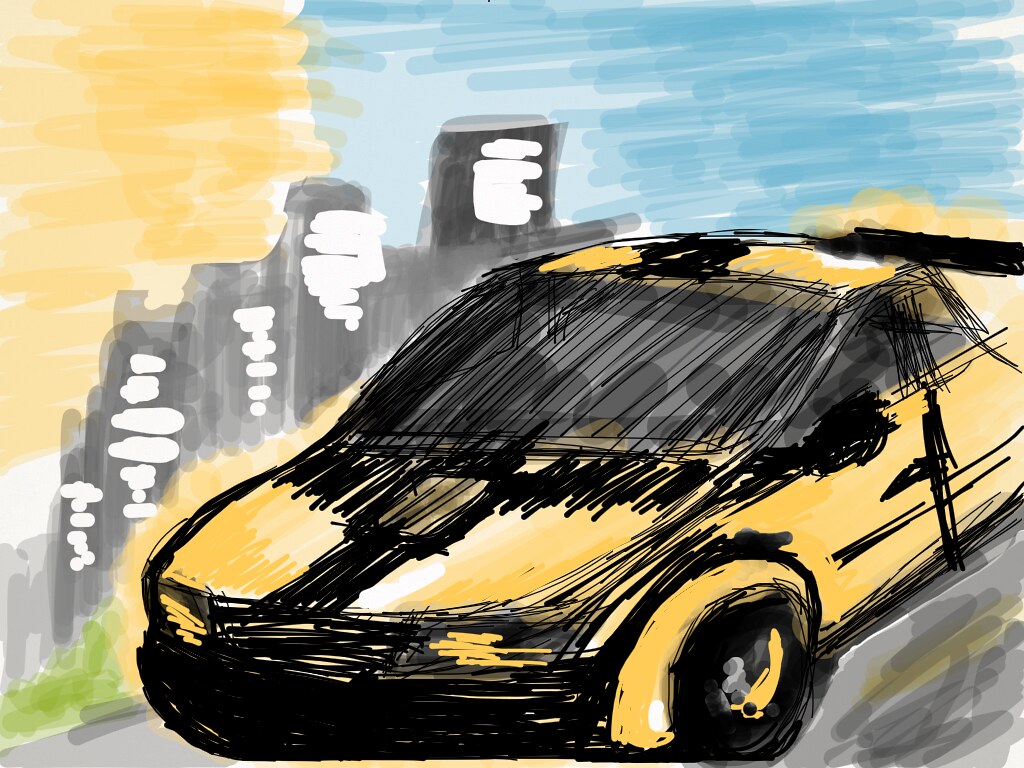This dynamic piece of hand-drawn artwork features a striking yellow sports car, adorned with vigorous black scribbles across various parts, including the hood and windshield. A black spoiler is prominently positioned at the back of the car, adding to its sporty appearance. The vehicle is set against an abstractly colored roadway, highlighted by a visible yellow line. A small patch of green grass adds a touch of nature to the scene. In the background, gray buildings with white scribbles enhance the urban setting, while a giant yellow sun radiates from one side, casting a warm glow. The sky is composed of light blue hues interspersed with darker blue streaks, evoking a sense of depth and movement. The windshield is decorated with multiple gray circular dots, and the car features prominent yellow headlights and black tires, with a particularly noticeable front tire. This imaginative and vibrant illustration captures a blend of realism and abstract creativity.